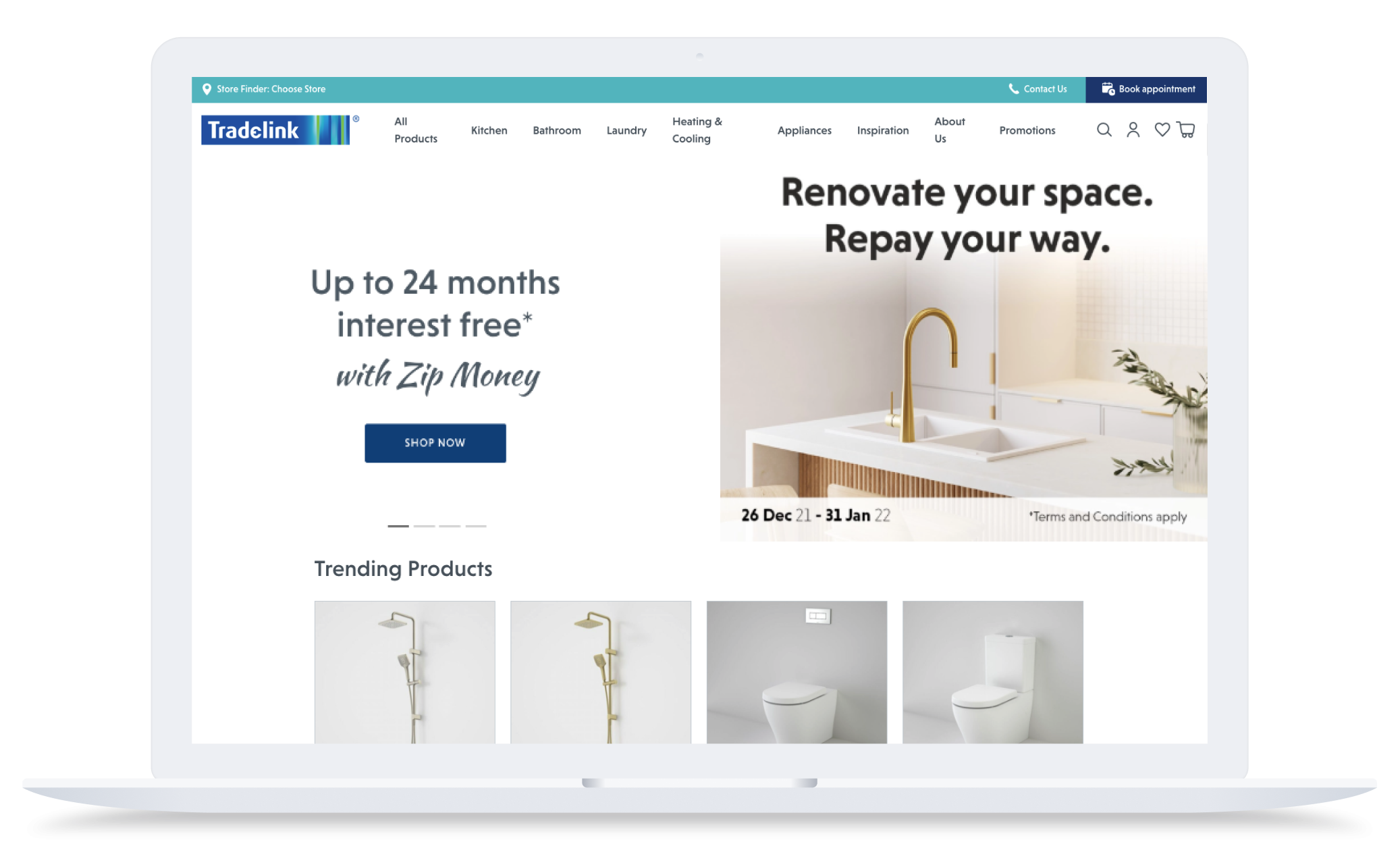The image depicts a promotional advertisement for the Tradelink website, prominently showcasing the Tradelink logo and name in the upper left corner. This advertisement encourages potential customers to take advantage of Tradelink's financing option, highlighting an exclusive offer: "Up to 24 months interest-free with zipMoney." Below this message is a call-to-action button labeled "Shop Now," inviting viewers to explore Tradelink's offerings.

Adjacent to this main promotional message is another advertisement stating, "Renovate your space. Repay your way. Terms and conditions apply." This further emphasizes the ease and flexibility of financing home renovations through Tradelink's partnership with zipMoney, a financing service that allows users to pay for their purchases interest-free over a specified period.

At the bottom of the advertisement, there's a bar displaying "Trending Products," suggesting that Tradelink offers popular items for bathroom renovations. The overall aim of the advertisement is to entice customers to renovate their bathrooms through Tradelink's website, providing the financial flexibility to do so with zipMoney’s interest-free credit program.